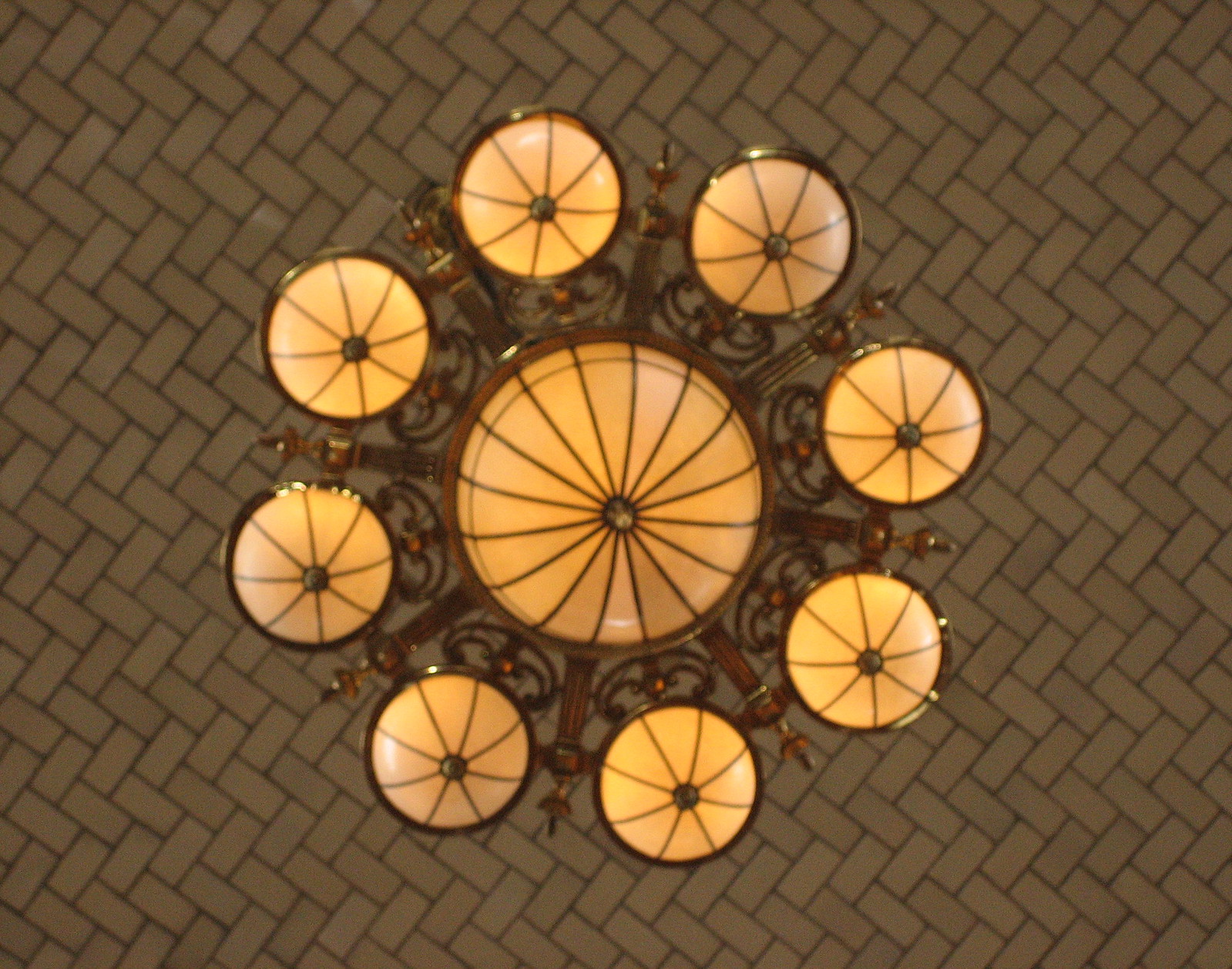The image captures an upward view of an elaborate chandelier, prominently centered though slightly off to the upper left. This chandelier boasts a large, amber-colored circular globe at its center, dissected into a dozen or more wedges by dark lines that give it a pie-like appearance. Surrounding this central globe are eight smaller circles, each about one-third the diameter of the main globe and similarly divided into eight wedge sections by dark lines. These smaller circles are intricately connected to the central globe by short, cylindrical fluted columns and ornamental C-shaped metalwork that seems reminiscent of wrought iron artistry. The chandelier's supporting brackets are a noteworthy brown hue adorned with various artistic shapes. The entire structure is lit, casting a warm yellow glow throughout. Above, the ceiling features rectangular tiles arranged in a complex herringbone pattern, creating a visually engaging zigzag effect that complements the chandelier's ornate design, making it a piece one might expect to find in a lavish restaurant or grand mansion.